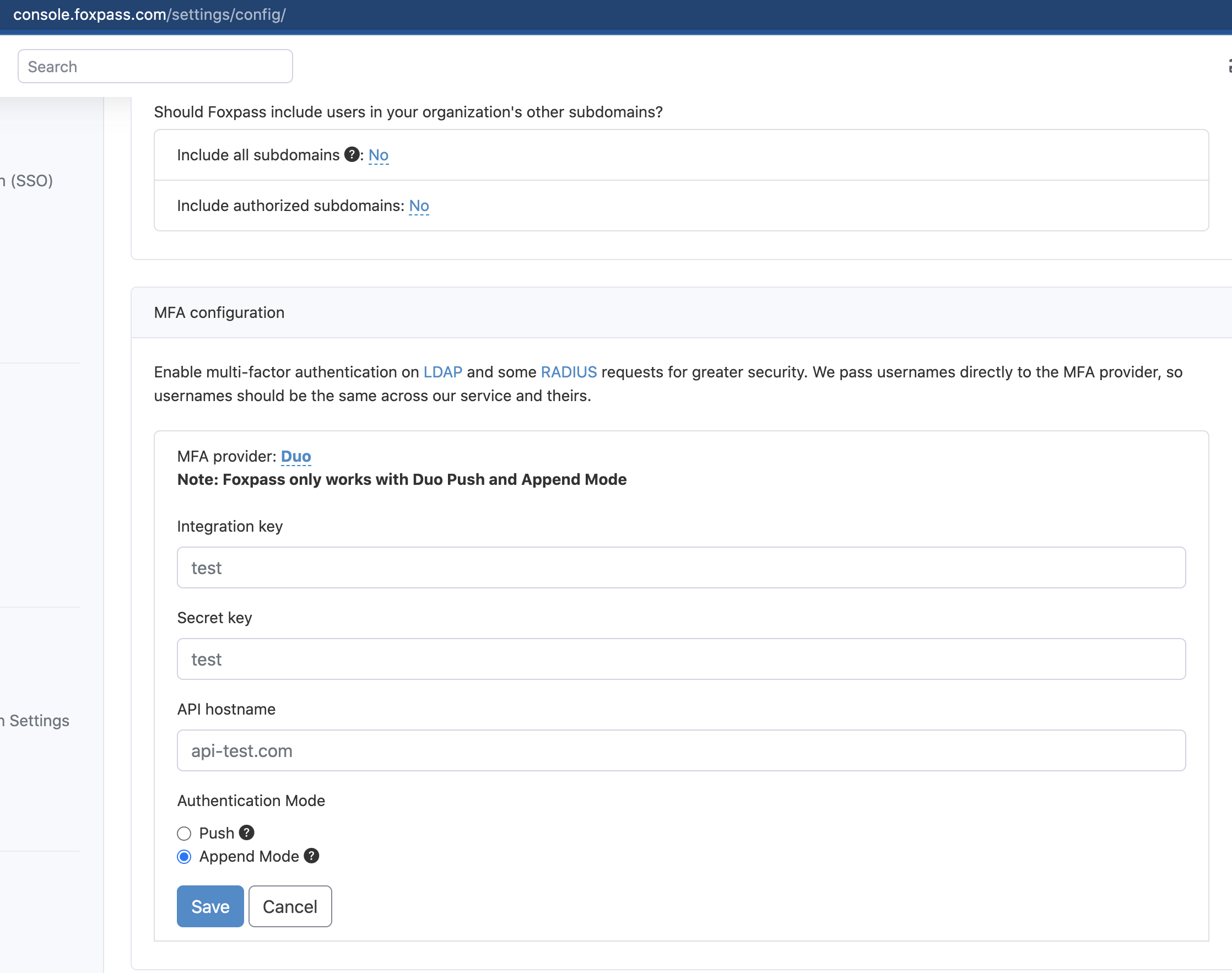The image shows the configuration settings page of FoxPass, a software or web application designed to enhance organizational security. The page URL is console.foxpass.com/settings/config. The settings being reviewed include integration with subdomains and multi-factor authentication (MFA) features. Specifically, there are options to include users from other subdomains within the organization, with current selections set to "No" for both "Include other subdomains?" and "Include authorized subdomains?" prompts. The section also addresses computer security through various text fields requiring input, such as the integration key, secret key, and API host name. These fields are essential for setting up MFA, which in this case utilizes Duo as the provider. It’s noted that FoxPass supports Duo's push and append modes for enhanced security during LDAP and other RADIUS requests.